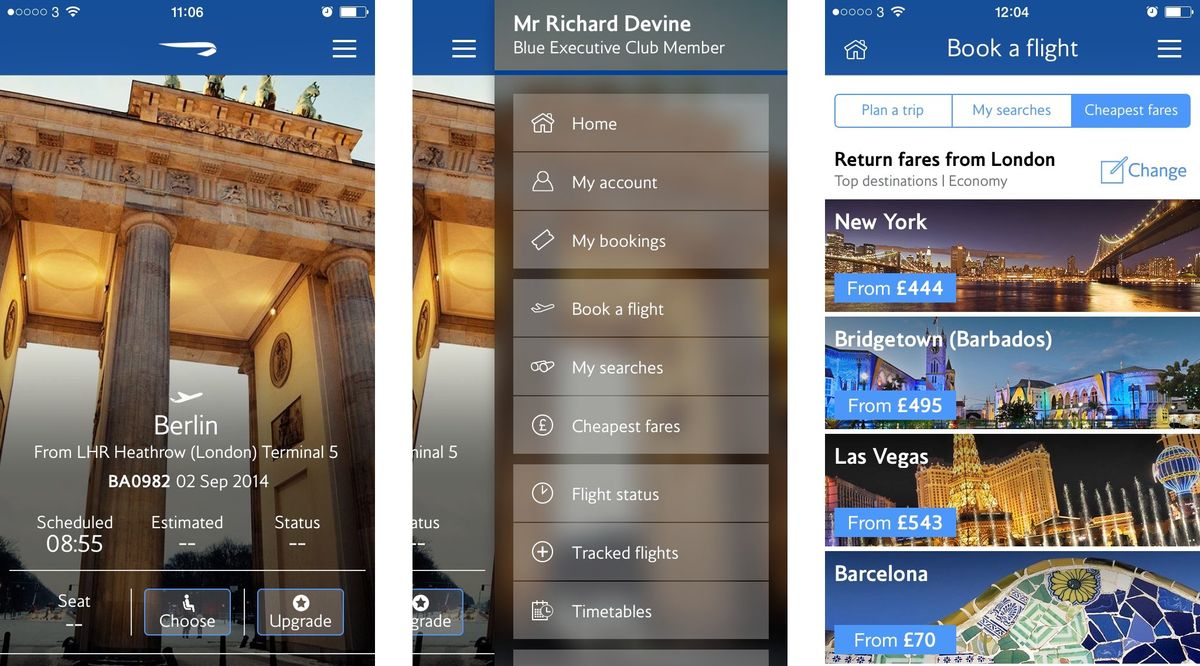This is a detailed screenshot of someone's travel dashboard, segmented into three distinct sections. 

On the left side, there's an image backdrop featuring a grand bridge with massive pillars and horse statues perched atop. Superimposed on this background is an icon of an airplane with the word "Berlin" written below in white text. The display shows scheduled and estimated times alongside a status update, accompanied by an icon indicating accessibility for handicapped individuals.

The middle section presents a gray header box with text that reads "Mr. Richard Devine, Blue Executive Club Member" in white. Directly beneath, a series of functional rectangles are arrayed vertically: the first displays a home icon and the word “Home,” followed by “My Account” with a generic icon, “My Bookings” with a ticket image, “Book a Flight” with an airplane icon, “My Searches,” and “Cheapest Fares.” Further options include “Flight Status,” “Tracked Flights,” and “Timetables.”

On the right, a series of cityscape images are arranged with corresponding text. One shows a bridge spanning over water labeled "New York" in white text. Another displays "Bridgetown, Barbados" against the backdrop of a prominent building. A third image depicts a brightly illuminated building with a fountain in front, captioned "Las Vegas."